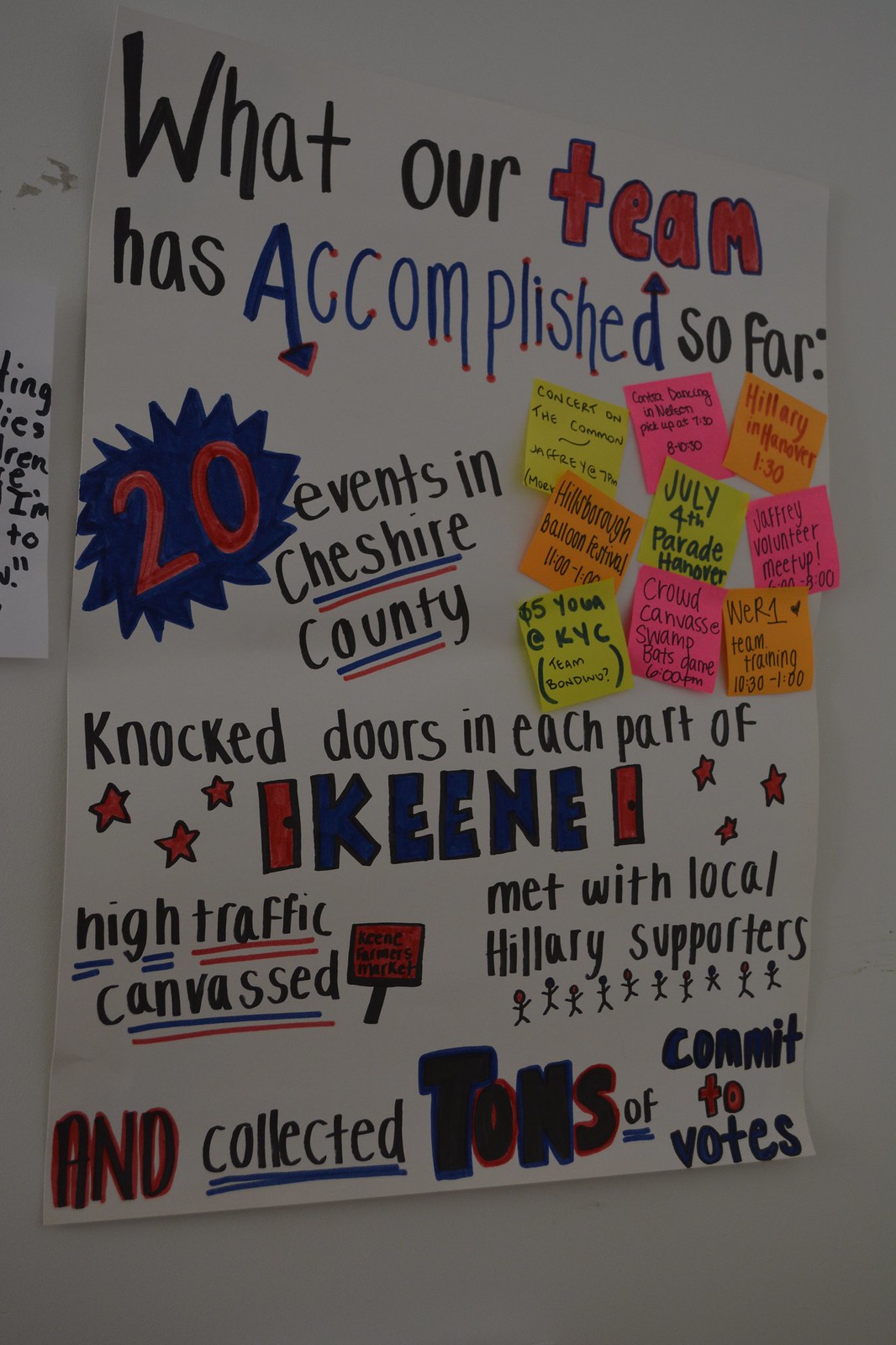The image depicts a handmade poster taped to a white wall, crafted on a white paper. The poster is titled "What Our Team Has Accomplished So Far" with the words written in a mix of black, red, and blue marker. Notably, "team" is highlighted in red and "accomplished" in blue. Beneath this heading, there is a prominent "20" written in red, outlined in blue, followed by the text "events in Cheshire County" in black. Adjacent to this, there are nine post-it notes detailing the various events. Moving down the poster, it lists their achievements: "knock doors in each part of Keene," with "Keene" in blue, "high-traffic canvassed," "met with local Hillary supporters," and "collected tons of commit-to-votes," with "tons" highlighted in blue and red. The poster also features illustrations of human stick figures, emphasizing the team's efforts and community engagement in their political canvassing activities.